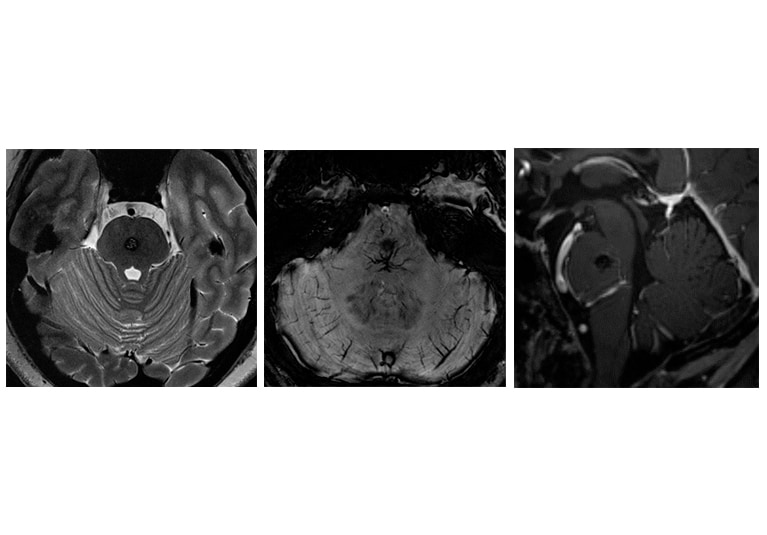The image comprises three horizontally arranged grayscale panels, each depicting different cross-sectional views from a medical brain scan, possibly an MRI or CT scan. The leftmost panel likely represents a top-down view of the entire brain within the skull, characterized by a white outer ring and concentric darker areas within. The central panel presents a closer view, potentially focusing on a specific brain region to examine any abnormalities. The rightmost panel is an even more magnified view, honing in on a particular area of interest that warrants further scrutiny. The images collectively illustrate a progression from a broader view to increasingly detailed scans, highlighting specific brain structures and potential areas of concern.